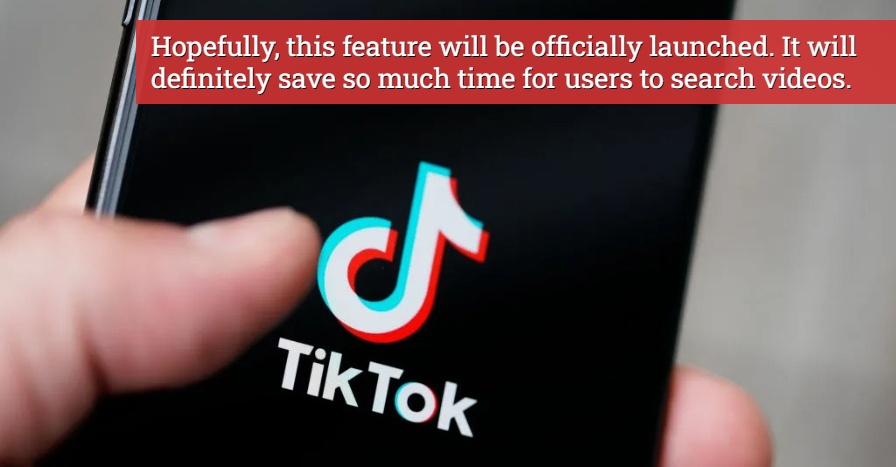A detailed close-up photograph prominently features a friend's hand holding a smartphone at an angle. The phone extends from the bottom edge of the image and is cut off at the top. Dominating the screen is the TikTok logo, characterized by its white icon accented with blue and red hues. Below the logo, the word "TikTok" is clearly visible. Positioned at the top of the screen within a distinct red box with white text, there is a hopeful caption stating, "Hopefully this feature will be officially launched. It will definitely save so much time for users to search videos." The overall composition makes the image appear almost like an ad for TikTok, effectively showcasing the platform's branding and the new feature announcement.